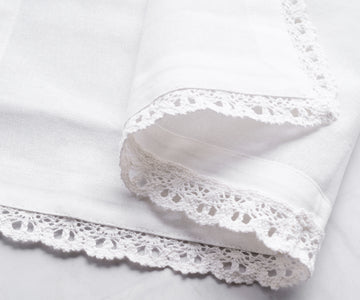This image showcases a carefully folded piece of white fabric, likely constructed of cotton, resembling either a kerchief or a tablecloth liner. It features a detailed, doily-like pattern with a lace trim that scallops around its edges, creating an intricate, crocheted finish. The fabric folds over onto itself twice at the top, presenting a thicker border and rounded center adorned with intricate circles. The material, reminiscent of a handkerchief or solid cloth doily, rests on a white surface, possibly a table. The image, in black and white, highlights the fabric's tight weave and the clean, refined appearance of both the fabric and the surface beneath it.